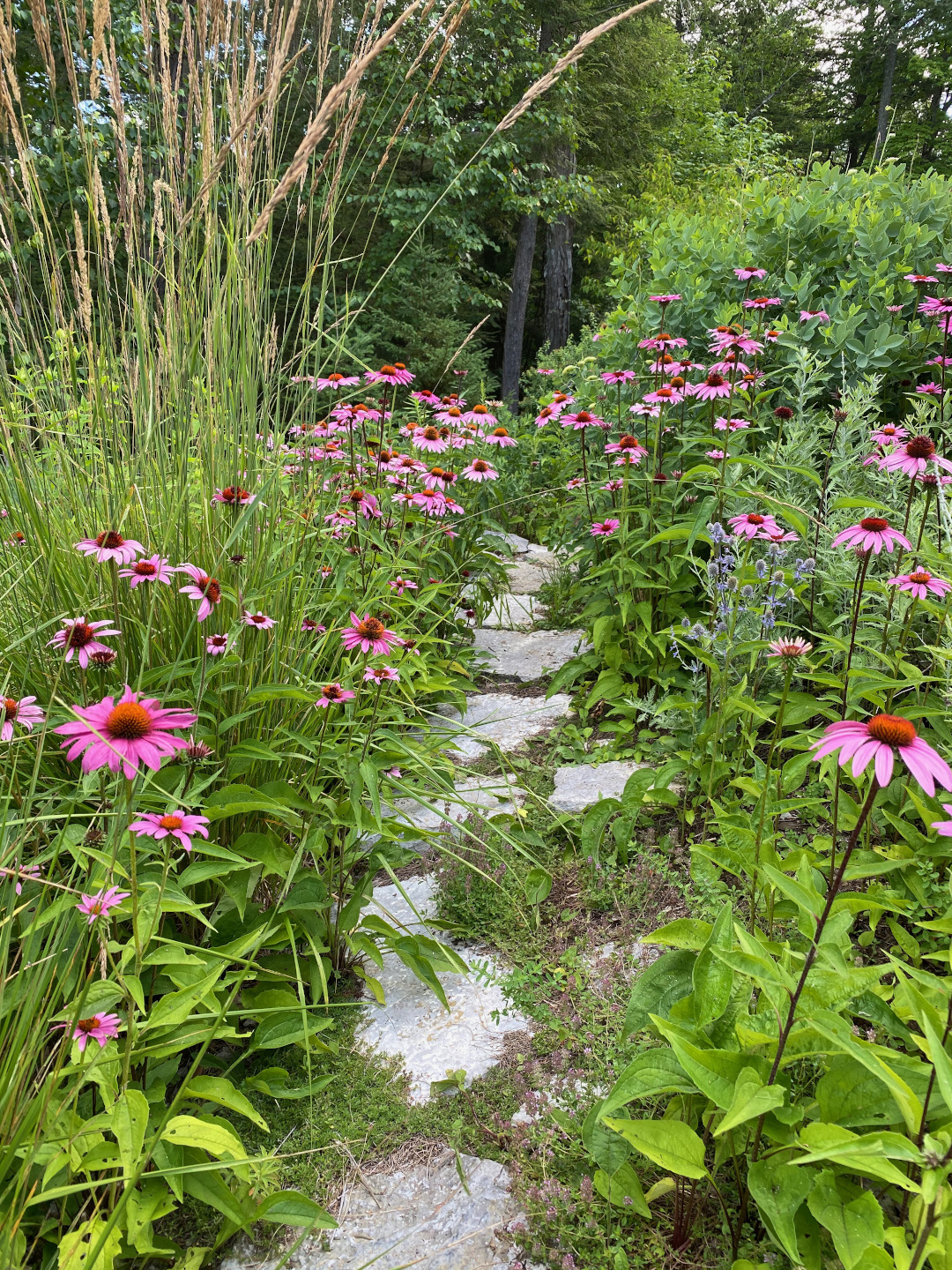The image depicts a picturesque walkway set with light gray stone tiles that leads into a forest, where the tall tree trunks are visible before giving way to a canopy of leaves. Flanking the path on either side are vibrant pink flowers with orange-red centers, likely daisies, creating a colorful, inviting border. The flowers are interspersed with various greenery, including large shrubs on the right, tall reeds on the left, and patches of grass sprouting through the stone walkway, contributing to a slightly overgrown appearance. The scene is bathed in soft, natural light on a somewhat cloudy day, accentuating the subtle shades of coral, green, and the earthy tones of the forest floor.